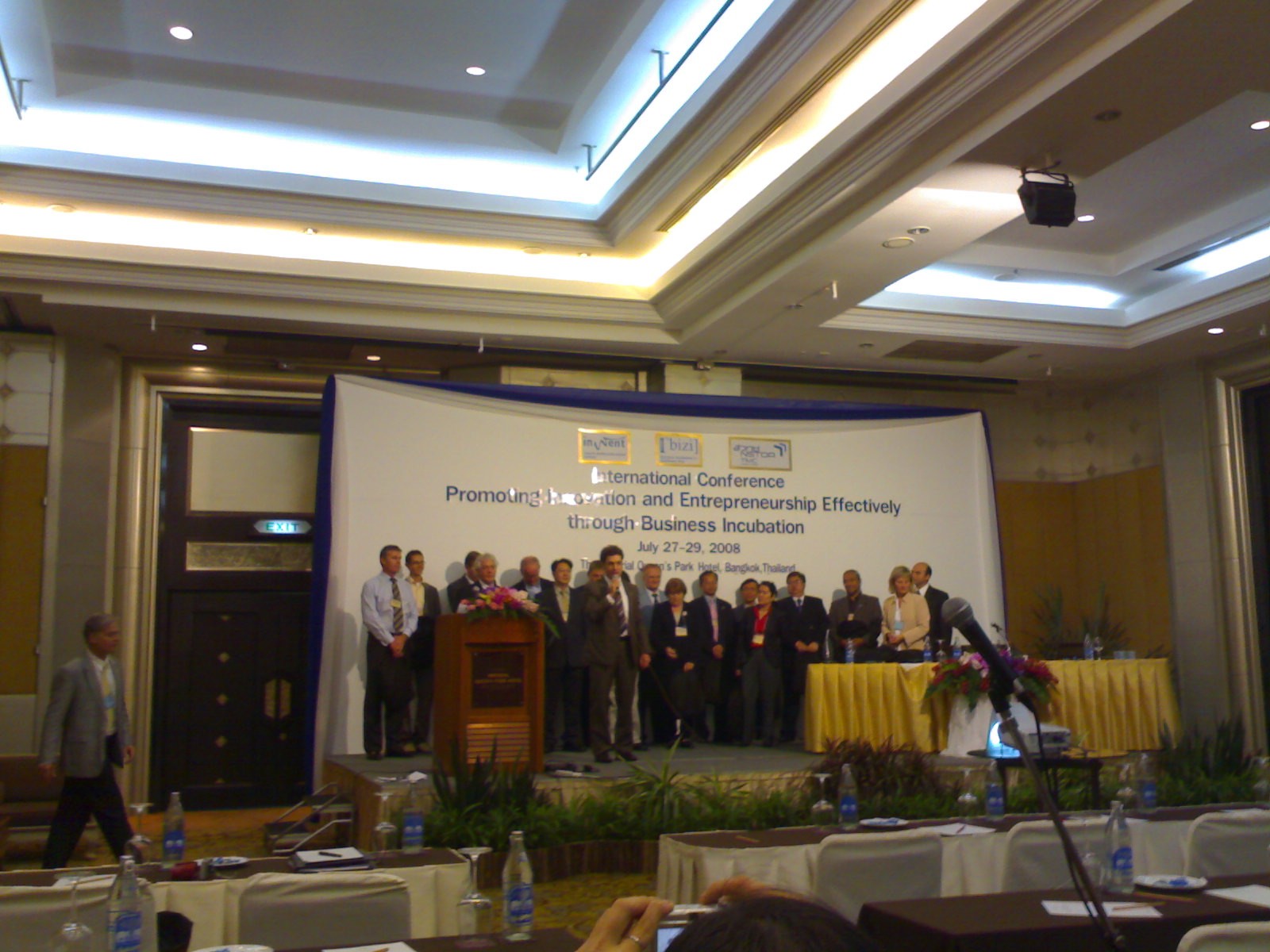Inside a grand ballroom-like meeting room adorned with cream-colored walls featuring elegant white tiling and softly glowing recessed lights in arched ceilings, an image captures a bustling scene at an international conference. On a stage set against a large, somewhat reflective white banner reading "International Conference Promoting Union and Entrepreneurship Effectively Through Business Incubation, July 27-29, 2008," a diverse group predominantly composed of older-looking individuals in business attire, likely of Asian descent, stands in formation. Towards the center of this group, a man wearing a brown suit speaks into a microphone, positioned next to a deep brown wooden podium adorned with a vibrant pink and white flower arrangement. To the right of the stage, a table draped with a golden yellow tablecloth adds a complementary touch. Scattered potted green plants add a touch of nature around the stage, while the tables in the audience, covered with white tablecloths and bottled waters, hint at the formal and organized nature of the event. Despite the image's slight blurriness, the solemnity and importance of the occasion shine through.